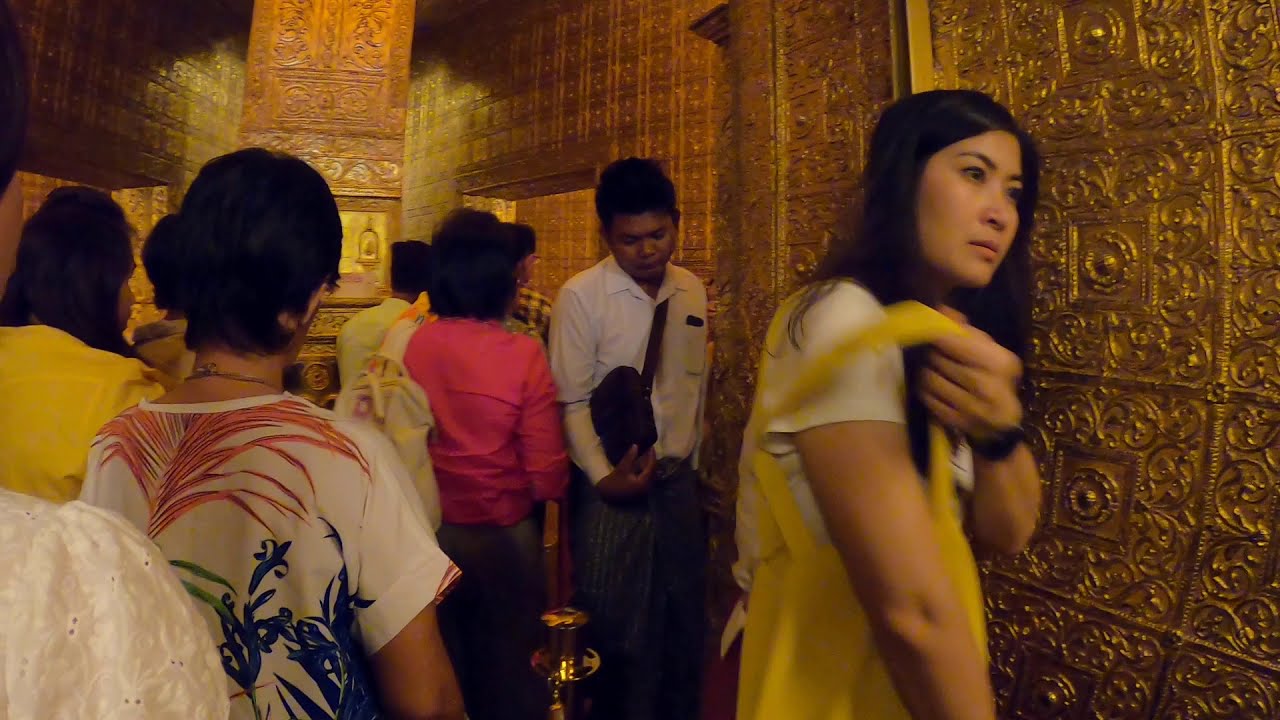In this richly detailed image, a group of six or seven people, predominantly women of Asian descent, are positioned in an opulent hallway adorned with intricate, gilded gold walls. The gold walls are deeply embossed with a square pattern that features curlicues, an additional square, and a circular medallion at its center, enhancing the grandeur of the setting. 

To the immediate right, a woman with long, dark hair wearing a white T-shirt adjusts the strap of her yellow canvas bag. She notably wears a black watch on her left hand. Slightly behind her, a man in a white button-up shirt with a black tie and dark pants looks towards the ground as he carries a black case. Walking alongside them on the opposite side of a barrier rope is another woman in a white blouse adorned with pink and blue leaf patterns.

At the center of the group, the path splits due to a robust column, which directs the flow of people. Among those walking away from the viewer, a woman in a pink sweater with a white backpack stands out. Nearby, a woman in a yellow top and dark pants navigates ahead. Most individuals in this scene are immersed in their own actions, contributing to the dynamic flow of visitors that move through this stunning temple-like venue.